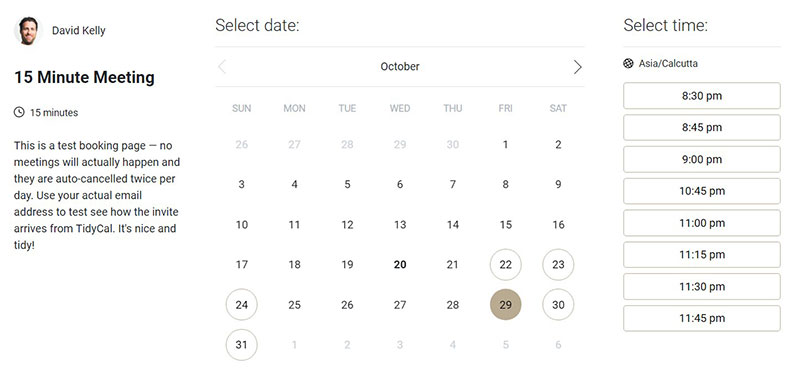The image showcases a calendar app interface, designed for booking and managing meetings. In the upper left-hand corner, there's a user profile icon displaying a white individual with a beard and short hair, named David Kelly. Below his name, a "15-minute meeting" is indicated alongside a clock icon. This appears to be a test booking page, where no actual meetings occur as they are auto-cancelled twice per day. Users are prompted to use their real email addresses to test how invitations from TidyCal are received.

Centrally, a calendar for October is displayed. At the top, there are greyed-out back and forward buttons. Several dates are highlighted with circles: the 22nd, 23rd, and 24th are simply outlined, while the 29th is filled in brown. The 30th and 31st also feature outlined circles. 

On the right, there is a "Select Time" section set to the Asia/Calcutta time zone. Times listed in brown-outlined rectangles with black text include: 8:30 PM, 8:45 PM, 9:00 PM, 10:45 PM, 11:00 PM, 11:15 PM, 11:30 PM, and 11:45 PM, likely corresponding to the highlighted date of the 29th. 

This interface is likely designed for users to become familiar with how the app functions.